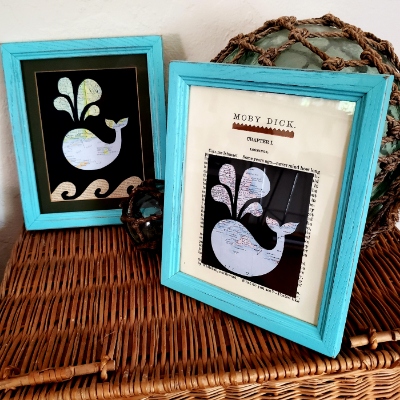The image depicts a wicker end table adorned with two framed pictures, both enclosed in light turquoise frames. The forefront picture features a whimsical whale set against a stark black background. The top of the image showcases the title "Moby Dick" in bold, uppercase black letters, separated from the rest of the composition by a brown, scalloped line. Below this, the tiny text "Chapter One" is visible, with a large, whimsical rendition of a whale emitting an exaggerated spout of water, almost reminiscent of golf club shapes.

To the left and slightly behind this main picture is another framed depiction of a whale. This second image repeats the whale motif with three small waves and a spout of water above its head, but it lacks any text. Just behind the leading picture lies a jute-covered glass ball, partially encased in a macrame netting. All these elements are carefully arranged atop the wicker chest, creating a cozy, nautical-themed display.